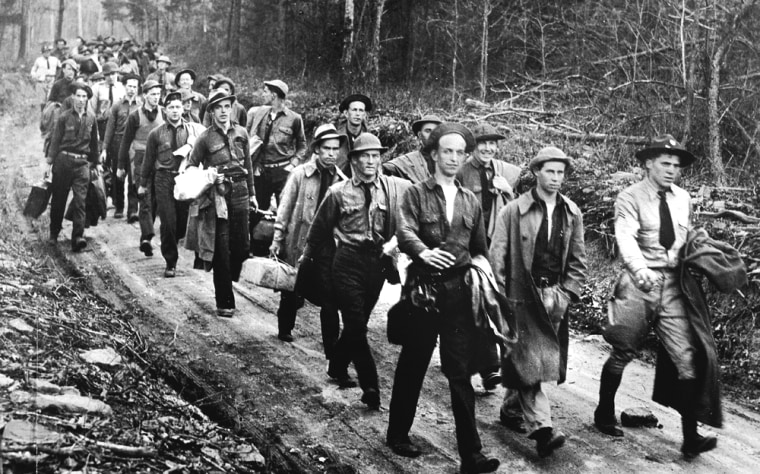This is a black-and-white photograph, likely taken in the 1940s or 1950s, featuring a large group of men, possibly numbering in the hundreds, marching down a dirt path that curves at an angle. The men, primarily white, are dressed in a mix of attire, including pants, long and short coats, some carrying their coats or bags, and nearly all wearing hats typical of the 1950s. The scene depicts mostly serious expressions, with only one man near the front showing a smile. The men are walking towards the bottom right corner of the image, and the pathway is bordered by a forested area with both standing and fallen trees. The trees seem to have been cleared close to the path, adding a sense of openness. The photograph captures both the clarity of the men at the front and the blurred motion of those further back, emphasizing the large scale of the group and their synchronized movement. The ambiguous mix of military and civilian appearances, especially with the leader in a white shirt, tie, and military-style hat, adds to the historical and possibly wartime context of the image.